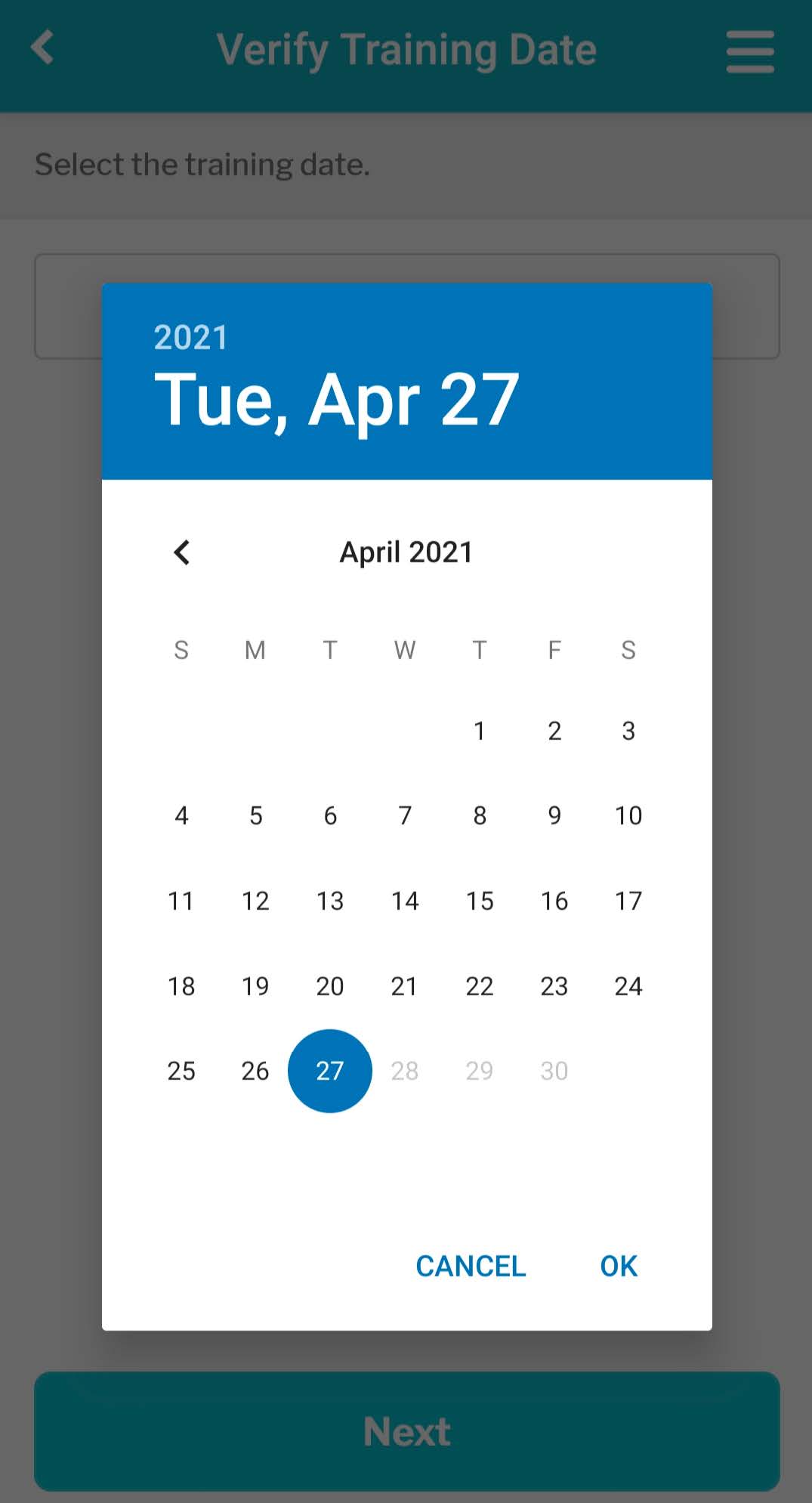A screenshot of a mobile calendar app interface is displayed. At the top of the screen, in white text, it reads "Verify training date" with horizontal bars next to it, indicating an interactive drop-down or menu option. Beneath this, it says "Select training date" in white font. Dominating the center of the screen is a calendar overlaid on the interface, showing the year 2021. The highlighted date is Tuesday, April 27th, prominently displayed in white text. The calendar grid is typical, with days and dates in black text. At the bottom, there's a prominent blue box labeled "Next," indicating a call to action for the user. The entire image is focused on the task of date selection within the app.